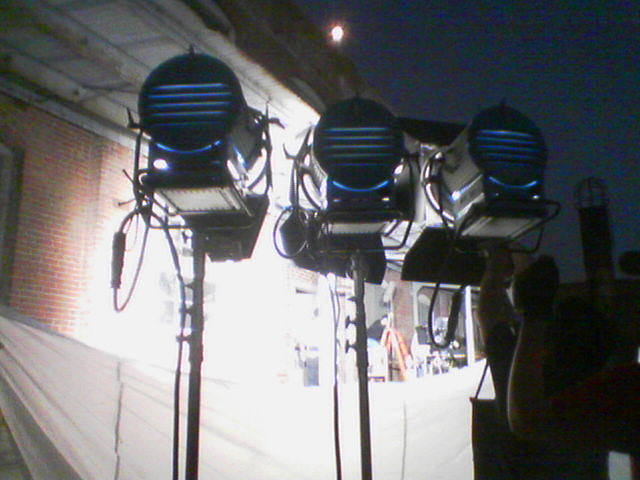The image appears to be an old, grainy photograph or a still frame from a video, characterised by a multicolored film grain and significant distortion. The photo captures a nighttime outdoor scene with the focus on three stage lights positioned centrally, mounted on long, thin black poles, each with circular fixtures featuring blue stripes. These lights are intensely bright, causing the surrounding details to blur and wash out. The lights are directed towards a brick wall on the left side of the image, indicating the side of a house or an apartment building. Above the wall, on the top left, the dark blue night sky is visible, with the moon glowing a soft yellow hue near the top center-right of the frame. There is a white tarp draped across the bottom half of the image, likely serving as a separator between the scene and the crew. In the bottom right corner, silhouettes of people are seen working on the light fixtures, though their features remain indistinguishable due to the darkness and blinding light. The overall composition suggests a film or theater production in progress.